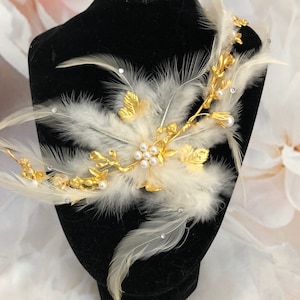The image displays a sophisticated piece of jewelry, prominently showcased on a classic black velvet mannequin neck, commonly seen in jewelry stores. The jewelry itself is intricate and eye-catching, featuring a combination of long, wavy white feathers and shimmering gold leaf inlays. The feathers fan out in various directions, adding a dynamic texture to the piece. Centrally situated within the feathers is a floral design composed of six pearls arranged in a flower pattern, with an additional smaller pearl situated on one side, emphasizing the detailed elegance. Interspersed among the feathers are small, delicate jewels that add a touch of sparkle. The backdrop accentuates the display, featuring a mix of pink and white gauzy fabric with a subtle floral pattern. This elaborate design, possibly a brooch or headpiece, occupies nearly the entire mannequin, showcasing its grandeur and ornamental sophistication.